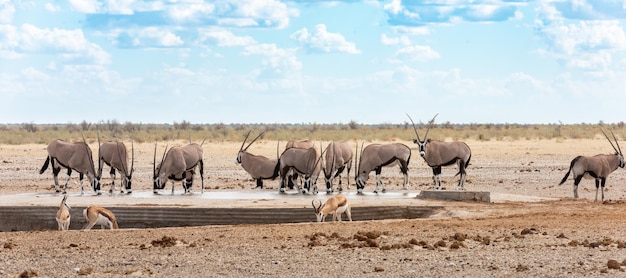In this color photograph, we observe a herd of antelope in a dry, barren landscape reminiscent of a desert, possibly in Africa. The flat terrain, under a sunny sky with light blue hues and scattered white clouds, highlights the arid conditions. The herd consists of twelve antelope, with nine adults and three lighter-colored juveniles, distinguished by their shorter horns and lighter tan fur with a darker stripe and white underbelly. The adults, predominantly gray with a white undertone and a thick black stripe, sport large, straight horns that extend prominently upward by their ears. The group is clustered around a sparse water source, either a small puddle or a dam, essential in such a desolate environment where vegetation is sparse and mostly brown. One adult antelope looks directly at the camera, adding a sense of connection to the scene. In the background, we can see a few dead-looking bushes, emphasizing the harsh, dry conditions.